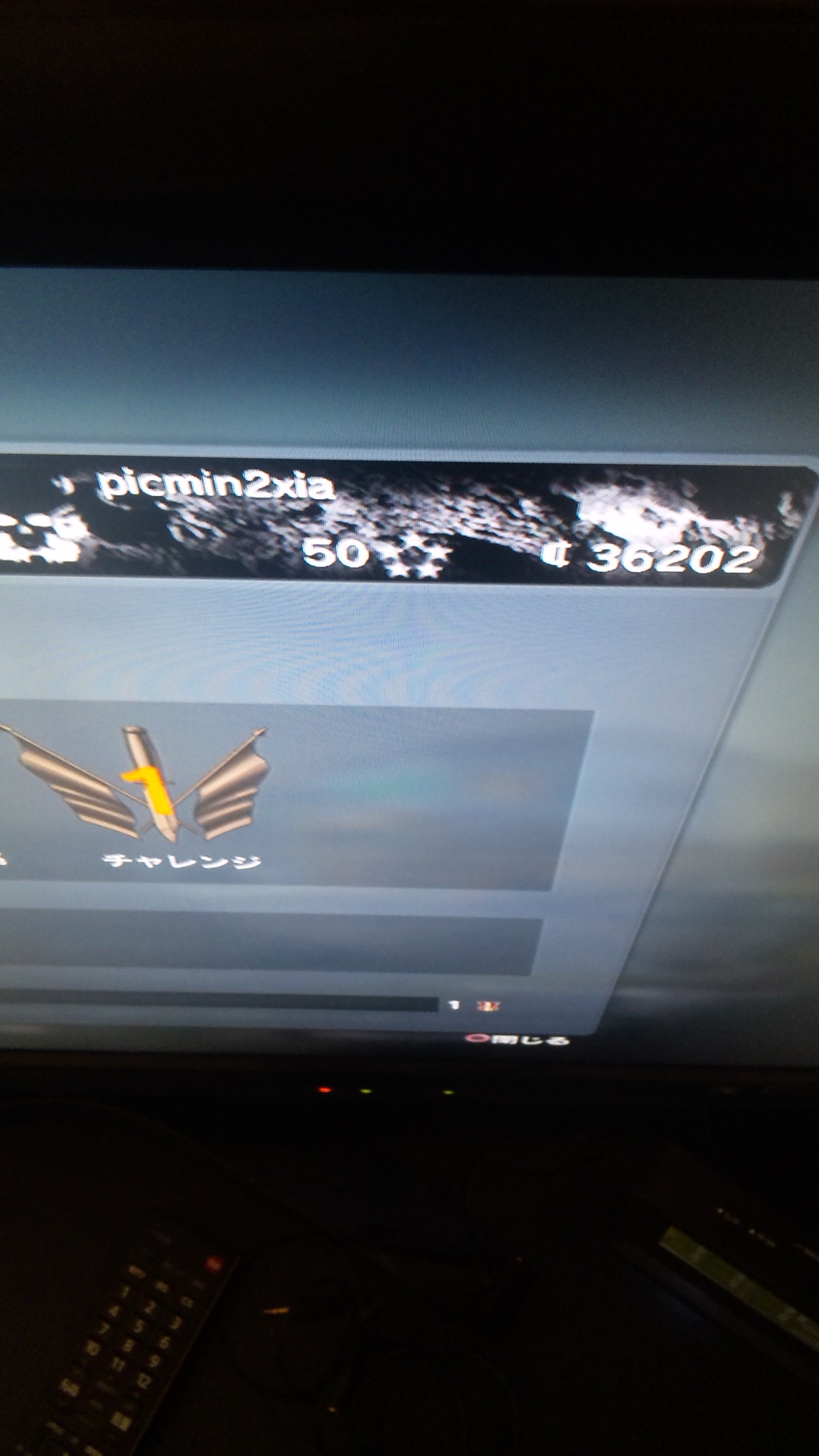The image depicts a high-angle view looking down at a TV or computer screen, possibly an idle screen for a video game. The scene is dimly lit, with most of the details centered on the screen and nearby objects. At the top of the screen, a black bar spans from left to right, beneath which is a purple bar. Written against the black bar in white letters is "P-I-C-M-I-N-2-X-I-A," accompanied by five white stars arranged in a pentagon shape. Off to the right, numeric details "3-6-2-0-2" are visible. The screen itself has a bluish-gray hue, featuring unidentified writing, possibly Arabic or Asian, alongside symbols or design drawings.

Just below this section, there appears to be a logo resembling an eagle with outspread wings, and three lights—red, green, and white—are visible under it. In the bottom left corner of the image, a remote control with a distinctive red power button can be seen, aimed away from the screen at an angle. To the right of the remote, there is a blurry, small electronic device, likely a router. The entire scene suggests this is an opening or waiting screen for a game, further implied by the gamer tag-like username and score displayed at the top.